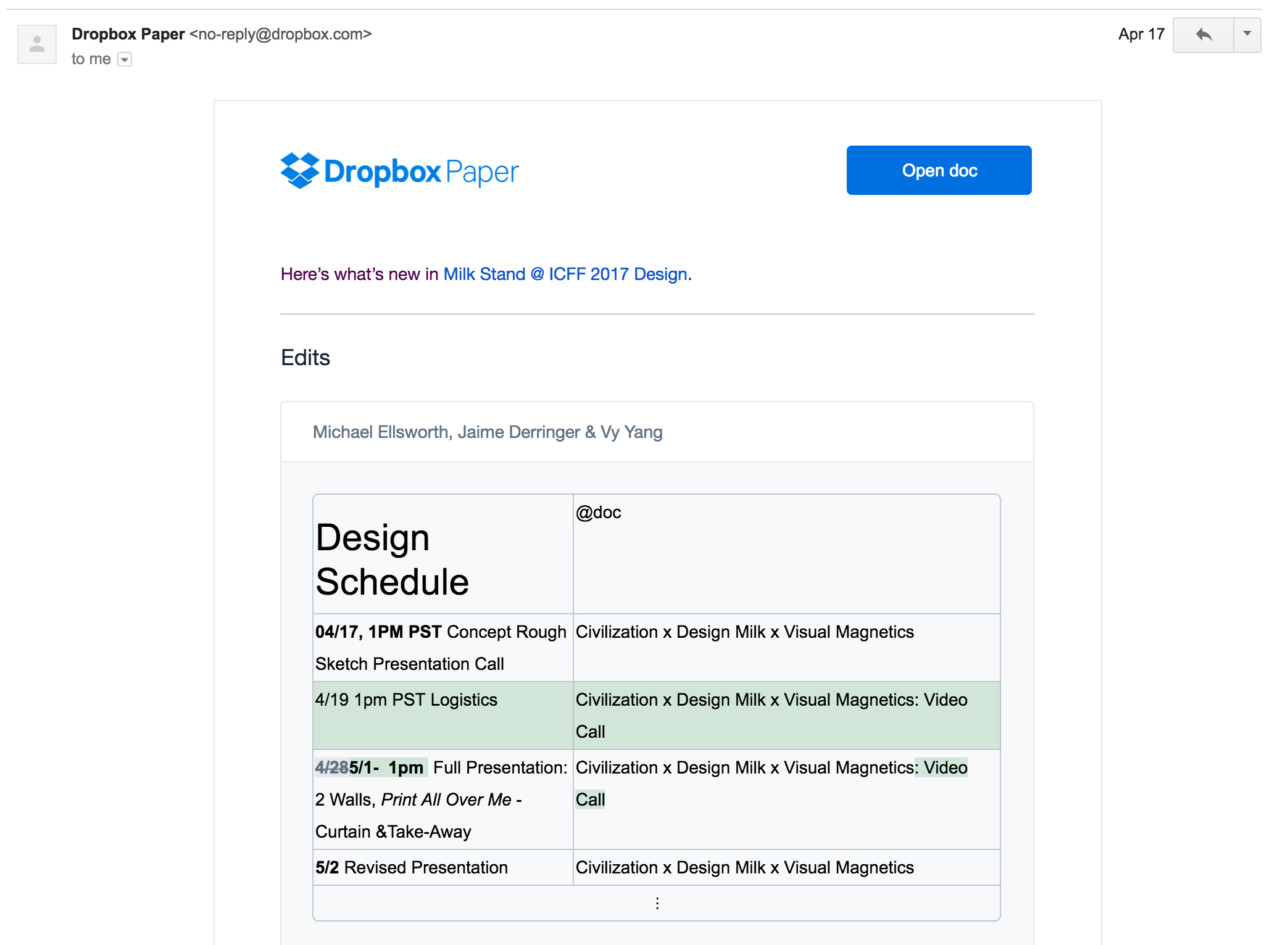Screenshot of a Dropbox Paper Document Summary Email

The screenshot showcases a webpage with a predominantly white background. In the upper left corner, the header "Dropbox Paper" is displayed in black font, followed by the email address "no-reply@dropbox.com" in brackets, and the recipient “to me” is indicated beneath it. On the upper right corner of the page, the date is noted as "April 17th."

A gray rectangle with a left-pointing arrow is visible just below this header section. The main content area of the screenshot features a white background with a central square outlined in black.

In the upper left corner of this square, there's an icon of an open blue box alongside the text "Dropbox Paper." On the upper right, a blue button with white text reads "Open doc." Below this button, a bold line of text states, "Here's what's new in Milk Stand at ICFF 2017 Design," followed by a horizontal black line.

Underneath this line, the heading "Edits" introduces another smaller square containing the names "Michael Ellsworth / Jamie Derringer" and "Vive Yang." Below this is a gray square featuring the text "design schedule at doc 04/17, 1 p.m. PST concept rough sketch presentation call."